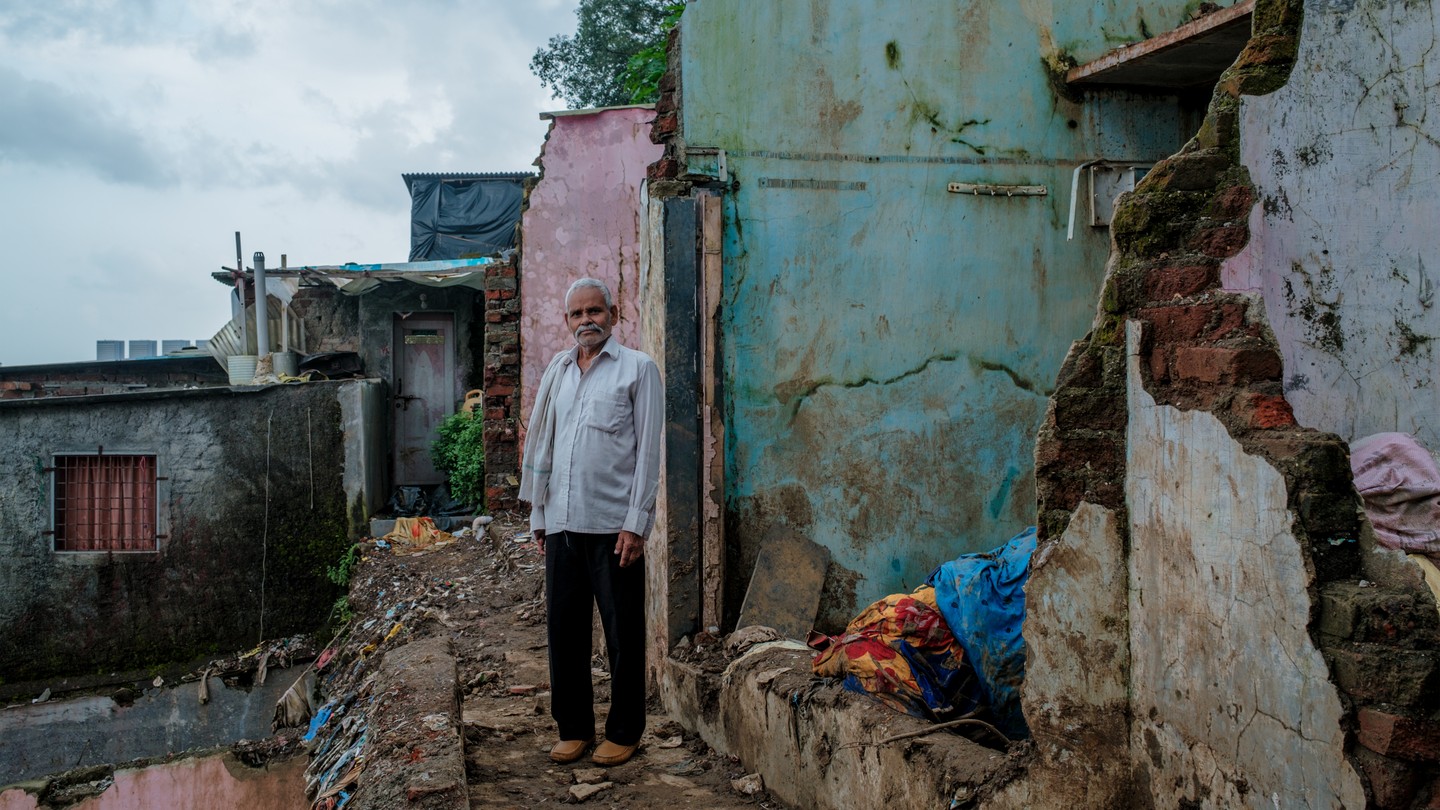The image depicts an older man standing amidst the remnants of a deteriorating cityscape, which appears unkempt and broken down, possibly due to a disaster. With short, bright white hair and a salt-and-pepper mustache paired with a patchy goatee, he looks to be in his 60s. Notably dressed in black pants, brown shoes, and a faded long-sleeved white or light-blue shirt, he carries a towel draped over his shoulder. The man stands in front of a wall painted in a faded pinkish rose color, with another bluish-teal structure to his left. Both structures show extensive damage, with parts of the walls missing, exposing red brick beneath the weathered, mildew-covered paint. The background reveals more similarly afflicted buildings with broken roofs, contributing to an overall sense of decay and hardship. Debris is scattered across the scene, underscoring the atmosphere of desolation in this sparsely populated or less dense city.